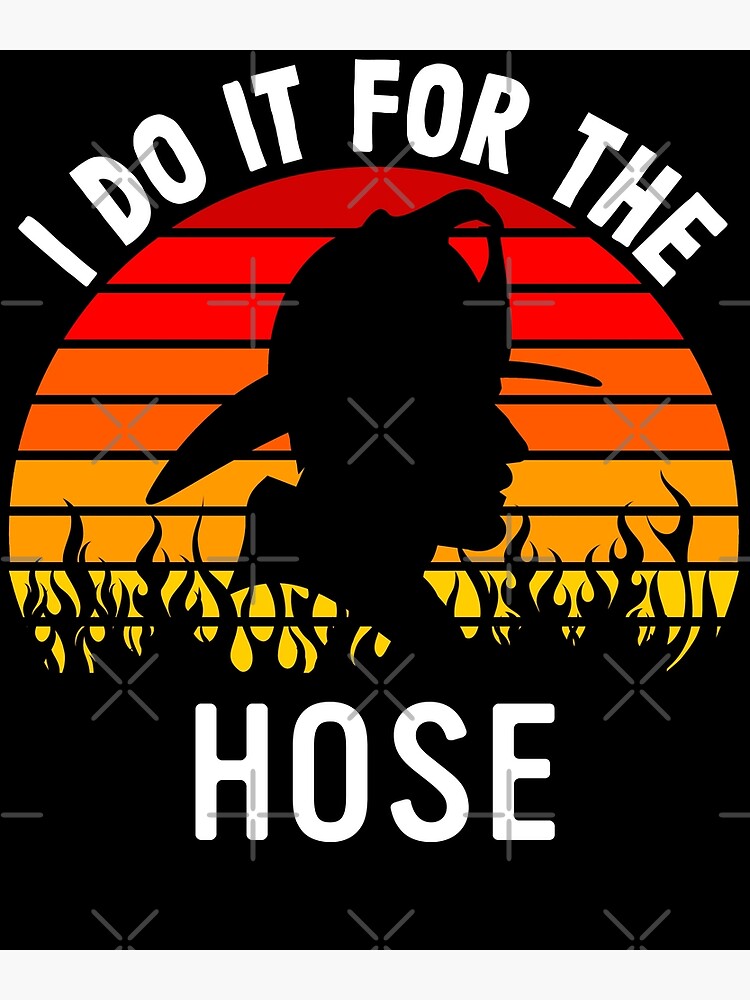The image is a computer-animated artwork set against a black background, adorned with gray X-shaped watermarks scattered throughout. Dominating the upper portion of the image, white text arches in a rainbow-like curve from one side to the other, stating "I do it for thee." Beneath this text, it reads "hoes," also in white. Central to the image is a multicolored circle resembling a sun or moon, with the bottom part not visible. The circle's gradient transitions from deep red at the top, through orange, to yellow at the bottom, divided by black lines. Flames depicted in black rise from the yellow section at the bottom of the circle. Superimposed against this vibrant background is the black silhouette of a firefighter, facing to the right, characterized by his collar and distinct fireman’s hat.